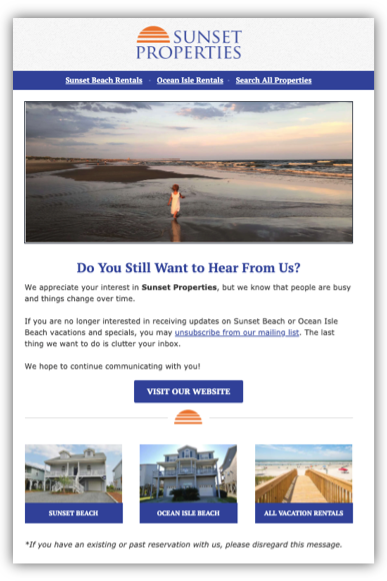At the very top of the image is a white background with some horizontal orange lines forming a half-circle. To the right of this design, the text "Sunset Properties" is displayed in blue. Below, a long navy blue horizontal line stretches across the width of the image, separating the content above from the following sections.

In the section beneath the navy line, there are three areas of interest, each with their text underlined: "Sunset Beach Rentals," "Ocean Isle Rentals," and "Search All Properties." 

Below these sections, an image captures a young girl in a white dress standing on sandy beach. The water is nearby, reflecting the dimming sky as evening approaches. The sky is a blend of pinkish-gray hues, scattered with clouds.

Following the image, in blue text, a question reads: "Do you still want to hear from us?" The subsequent text, in black, expresses appreciation for the viewer's interest in Sunset Properties, acknowledging that people’s interests and schedules may change. It provides an option to unsubscribe from future mailings if it is no longer desired, with "unsubscribe from our mailing list" underlined in blue. A concluding sentence reassures that the last thing Sunset Properties wants is to clutter anyone’s inbox, hoping to maintain communication with those interested. 

A blue box labeled "Visit Our Website" invites viewers to explore further. 

Towards the bottom, the image features three squares, each displaying different pictures of beach houses. The last square includes an image of a long walkway leading to the sandy beach and ocean.